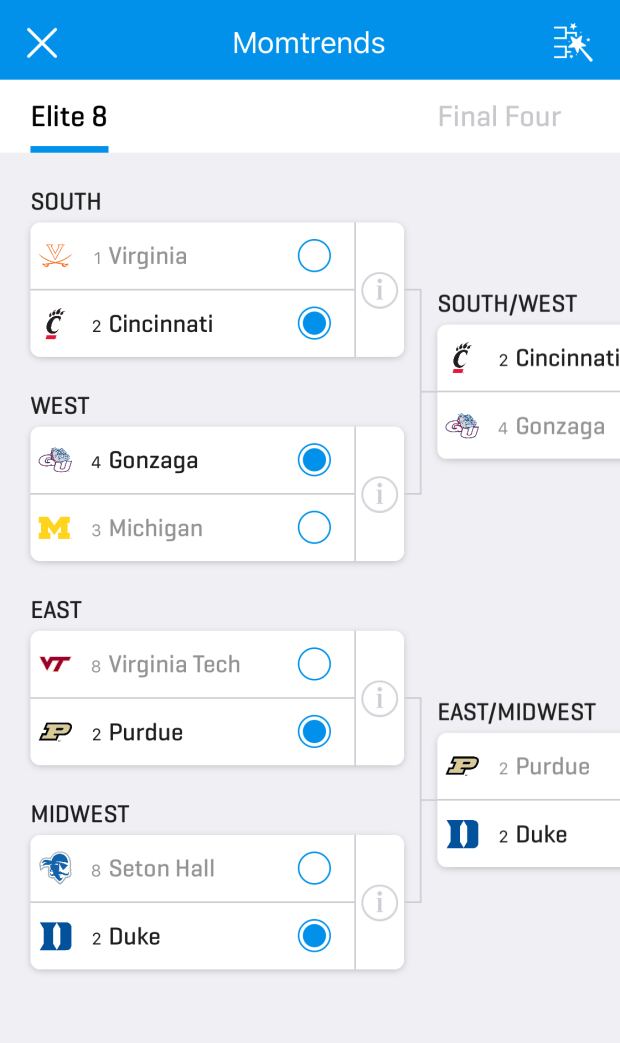This image features the "Mom Trends" app interface. Prominently displayed at the top center is the app's title, "Mom Trends," in white font with a capitalized "M" and "T," set against a blue banner. On the upper left-hand corner of the banner, there is a white 'X' icon used to close the screen. On the upper right-hand corner, there is an icon resembling a wand, also in white.

Just below this header, the tab labeled "Elite 8" is highlighted, indicating its active status. The main section of the display showcases a tournament bracket, reminiscent of a March Madness style chart. The chart is divided into four sections: South, West, East, and Midwest. Each section lists pairings of teams as follows: South features Virginia and Cincinnati; West includes Gonzaga and Michigan; East has Virginia Tech and Purdue; and Midwest lists Seton Hall and Duke.